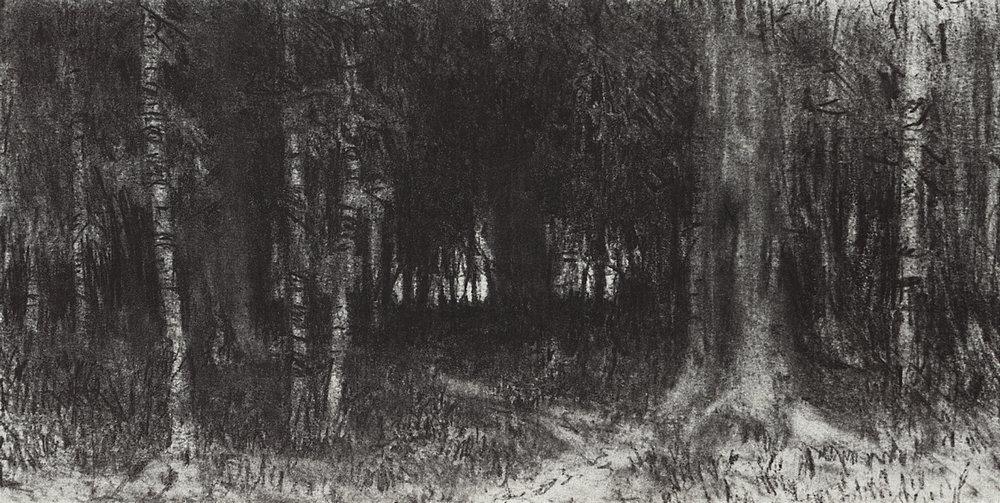This detailed charcoal artwork on white paper captures a dense, somber forest scene in a black, white, and gray palette, emphasizing the intricate tree trunks. The artist employed both heavy and light shading to convey depth and create middle ranges of gray, with patches of soil and sparse grass peeking through the forest floor. The image features a mix of birch, aspen, and pine trees, whose tops and foliage are largely out of frame, allowing the textured trunks to dominate the composition. Fleeting glimpses of sky, rendered as white spaces, contrast with the dark, dense undergrowth and branches, enhancing the artwork's serious and contemplative mood. The piece measures approximately eight to nine inches wide by five inches tall, lacks any signature or date, and presents no border or text.